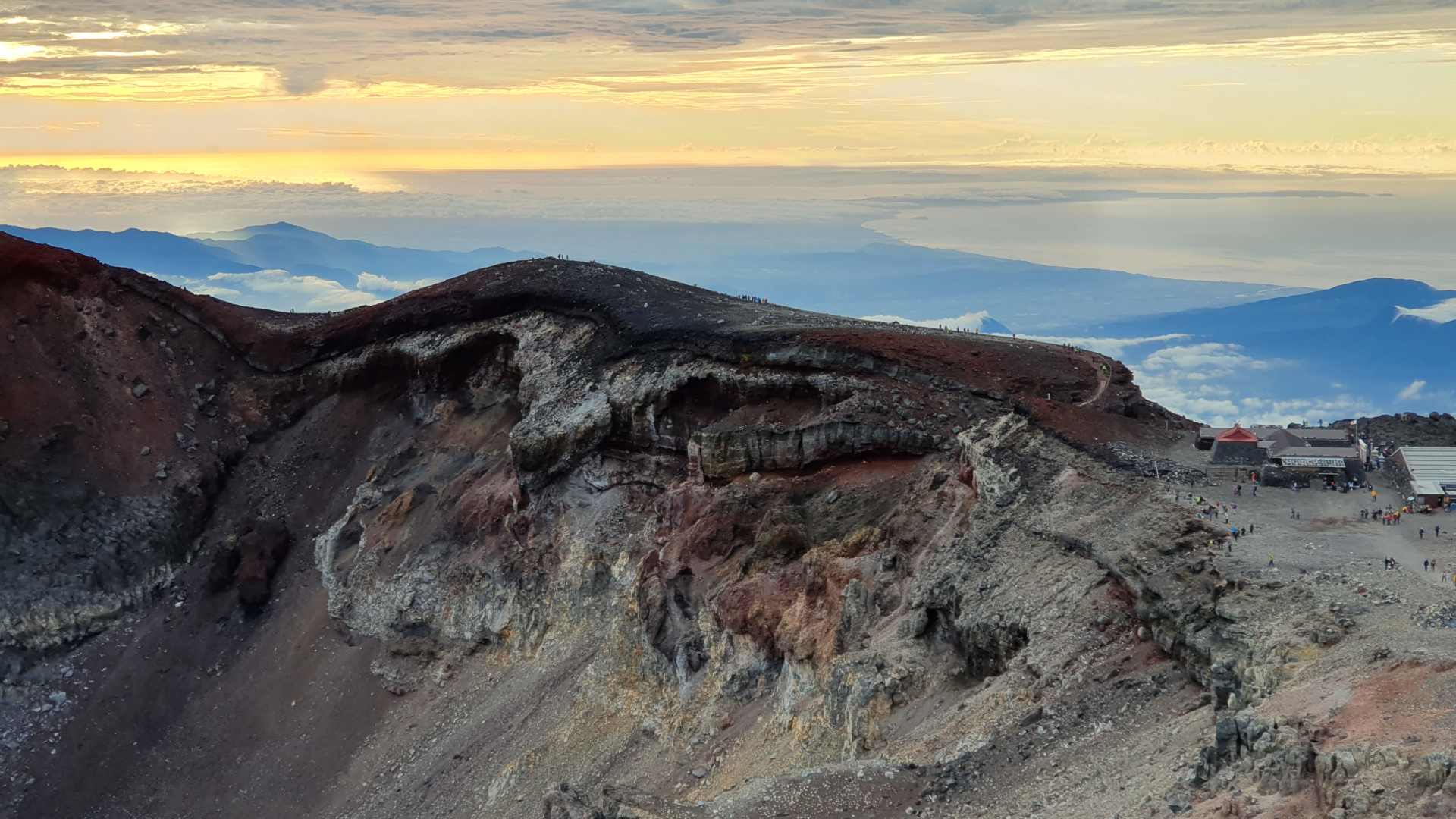The image captures a dramatic outdoor scene featuring a high mountainside near the ocean or beach, bathed in the golden hues of a sunset. The sky is illuminated with vibrant orange and golden yellow tones as the sun dips below the horizon, surrounded by numerous clouds both above and below the mountaintop. The crest of the mountain appears smooth, contrasting with the jagged, craggy landscape that drops steeply on one side. In the lower part of the image, hazy blue mountains loom under a dense layer of clouds, adding depth and scale to the scene.

The mountaintop itself is bustling with activity, dotted with many people, giving it the appearance of a popular tourist attraction. There are several buildings visible, including a tent with a distinct red pointed roof, and people are seen milling about, clearly enjoying the panoramic views. This rocky, sandy-looking mountainous mass, with its dramatic topography and scenic backdrop, serves as a picturesque and inviting destination for visitors.